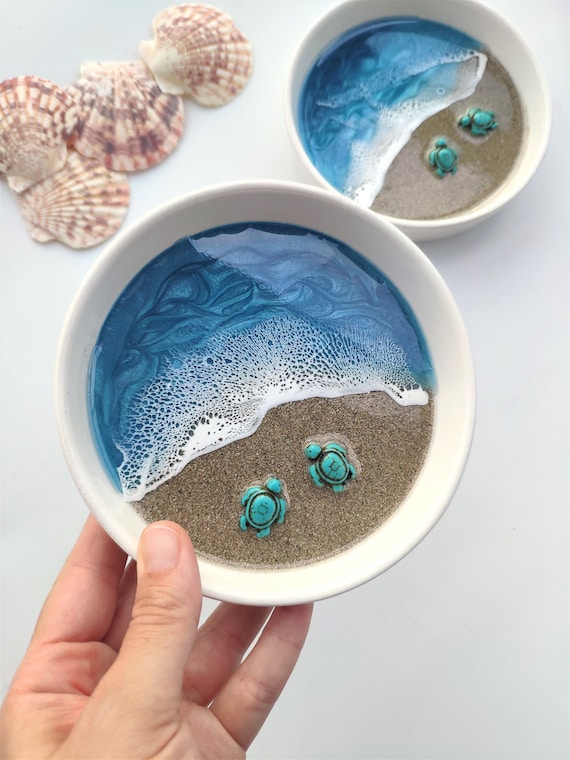This photograph showcases an intricately designed piece of art resembling a small, shallow bowl held by a white man's left hand. The bowl, which could easily be compared to a cereal bowl, contains a detailed miniature beach scene. The bottom of the bowl is filled with gray sand, artistically arranged to mimic a shoreline. Emerging from the sandy part are two little green turtle figurines, adding a touch of realism to the setting. The scene transitions seamlessly into a painted or glazed representation of the ocean, featuring blue waves that culminate in sea foam as they approach the shore. This artistic interpretation of the ocean occupies about half of the bowl's interior, creating a striking contrast with the sandy beach. In the upper right corner of the image, an identical bowl with a similar beach design is visible on the table. Additionally, the table features four seashells in shades of white and burnt red in the top left corner, contributing to the nautical theme. This unique and visually captivating artwork is unlike anything commonly seen, sparking curiosity about the techniques used in its creation.